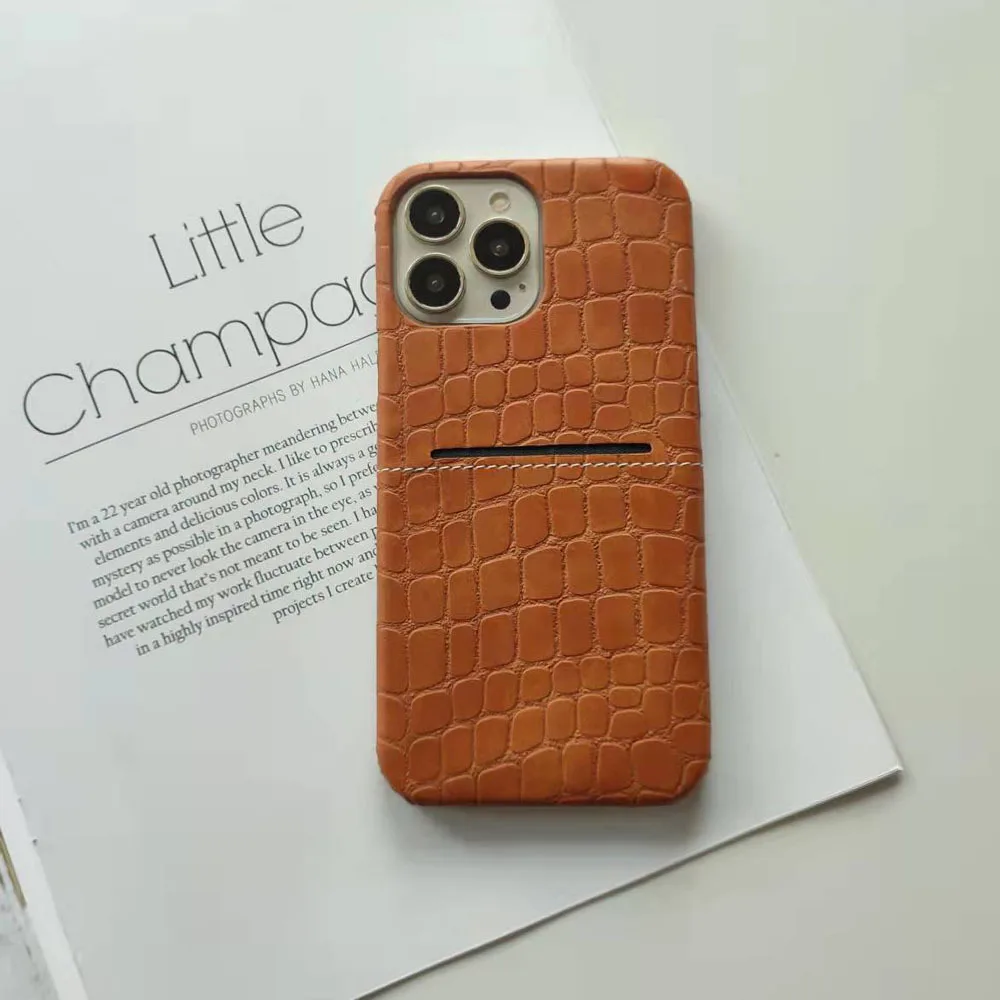The image features an iPhone lying face down with its distinct three cameras prominently visible. The phone is encased in a tan-colored cover that mimics alligator skin, complete with small, square scales of varying sizes. A mysterious black slot is situated in the middle of the cover. The phone rests on a slightly angled white piece of paper, which is mostly obscured by the phone. Legible sections of the text on the paper include "Little Champ" and a description by a photographer stating, "I'm a 22-year-old photographer meandering with a camera around my neck." The setting appears to be indoors on a table, and the overall image color palette includes shades of tan, gray, black, and white.